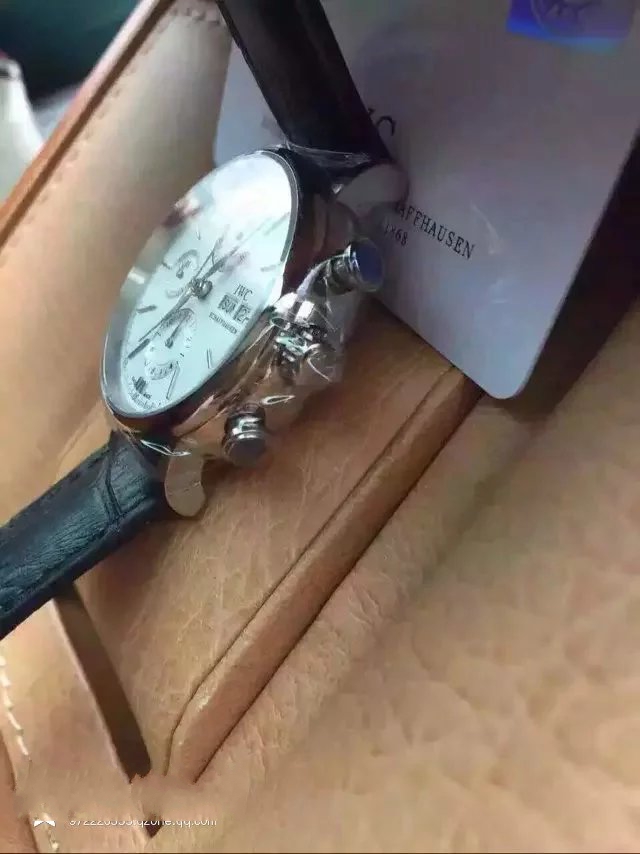This image, despite its low resolution and significant blurriness, depicts a wristwatch prominently centered. The watch band, visible on both sides, is black with a leather-like texture. The casing of the watch is silver and features three circular knobs on its right side. Though the image is fuzzy and somewhat pixelated, the face of the watch appears white with silver hands. There is also some indistinguishable white writing in the bottom left corner of the image, which is too small and blurry to read.